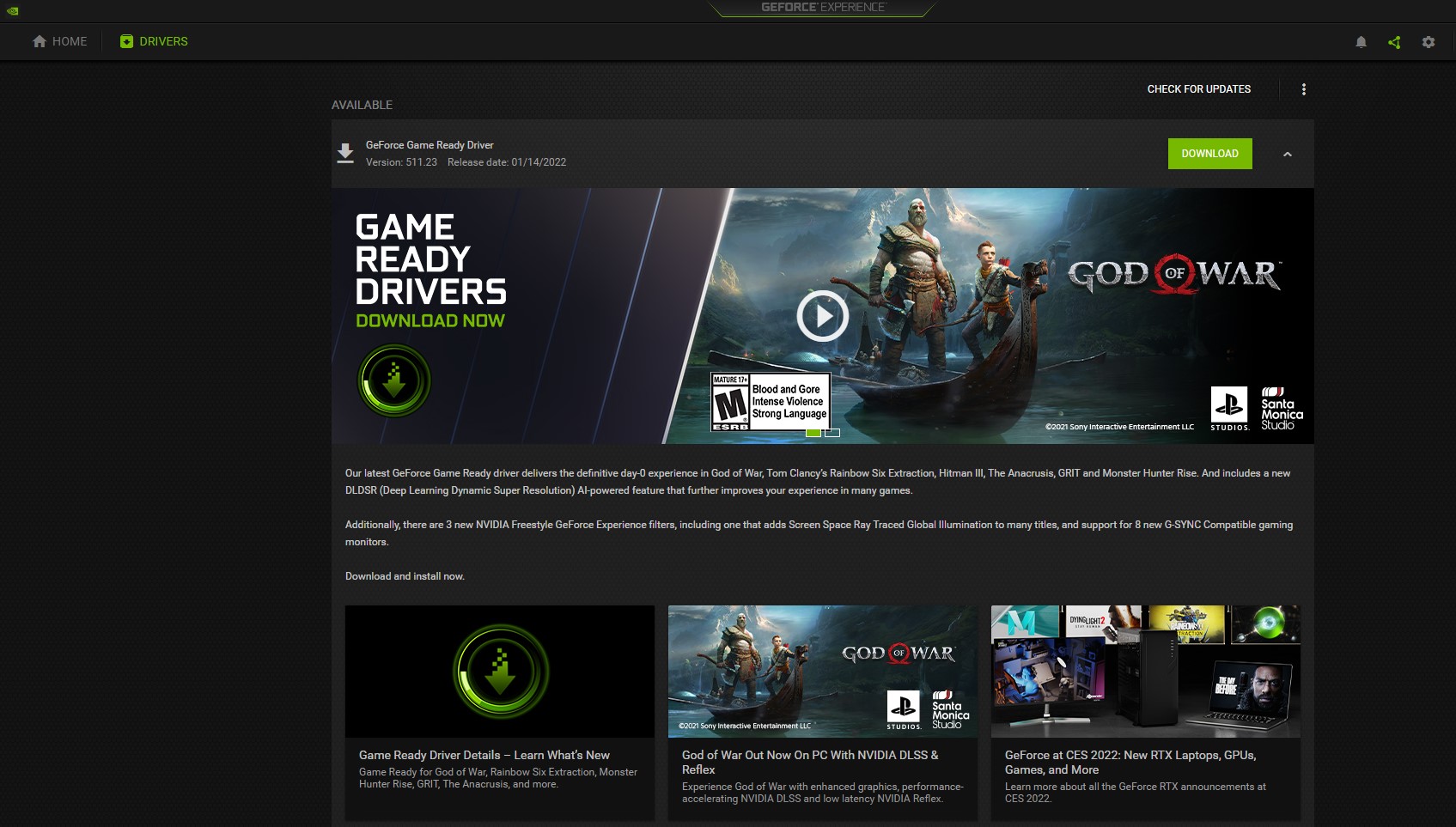The image displays a computer screen showcasing the game "God of War." In the upper left-hand corner, there is a black background featuring text that reads "Home" and "Drivers." Below this, it states, "Available check for updates." The central image highlights a large man, dressed as a Viking warrior, wielding a massive axe. In front of him stands a young boy holding a stick, both situated on a boat in a dark, shadowy location. 

The text on the screen includes:
- "Game Ready Drivers"
- "Download now"
- "God of War, blood and gore, intense violence, strong language, Santa Monica Studio"
- "Our latest GeForce Game Ready Driver delivers the definitive Day Zero experience in God of War, Tom Clancy's Rainbow Six Extraction, Hitman 3, The Anacrusis, Grit, and Monster Hunter Rise and includes a new DLDSR (Deep Learning Dynamic Super Resolution) AI-powered feature that further improves your experience in many games."

Additionally, there is more accompanying text and a smaller, similar picture of the man and boy on the boat positioned below. A green circle with a downward-pointing arrow and the words "Download now" in green are also visible.